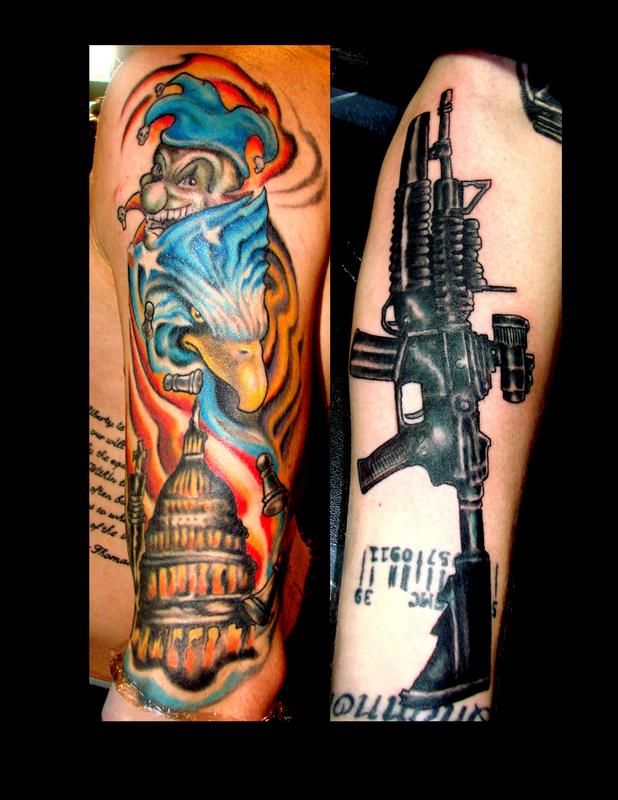The photograph features two tattooed arms set against a completely black background, centered in the middle of the image. The arm on the right displays a detailed tattoo of a black automatic rifle, possibly an AR-15, with a scope pointed up towards the person's shoulder. Just below the rifle is a barcode tattoo along with some unreadable text. The left arm showcases an elaborate, vivid tattoo starting with a sinister-looking court jester at the top, adorned in a blue and white jester's hat with tassels. Below the jester's malevolent grin is the head of a blue eagle, white feathers starkly contrasted with blue tones, evoking the American flag with red and white stripes and white stars swirling around it. Continuing down, the tattoo depicts the dome of the U.S. Capitol building, illustrated in hues of yellow and orange, with flames and a small chess pawn located at the lower part of the design. Both tattooed arms belong to white individuals.